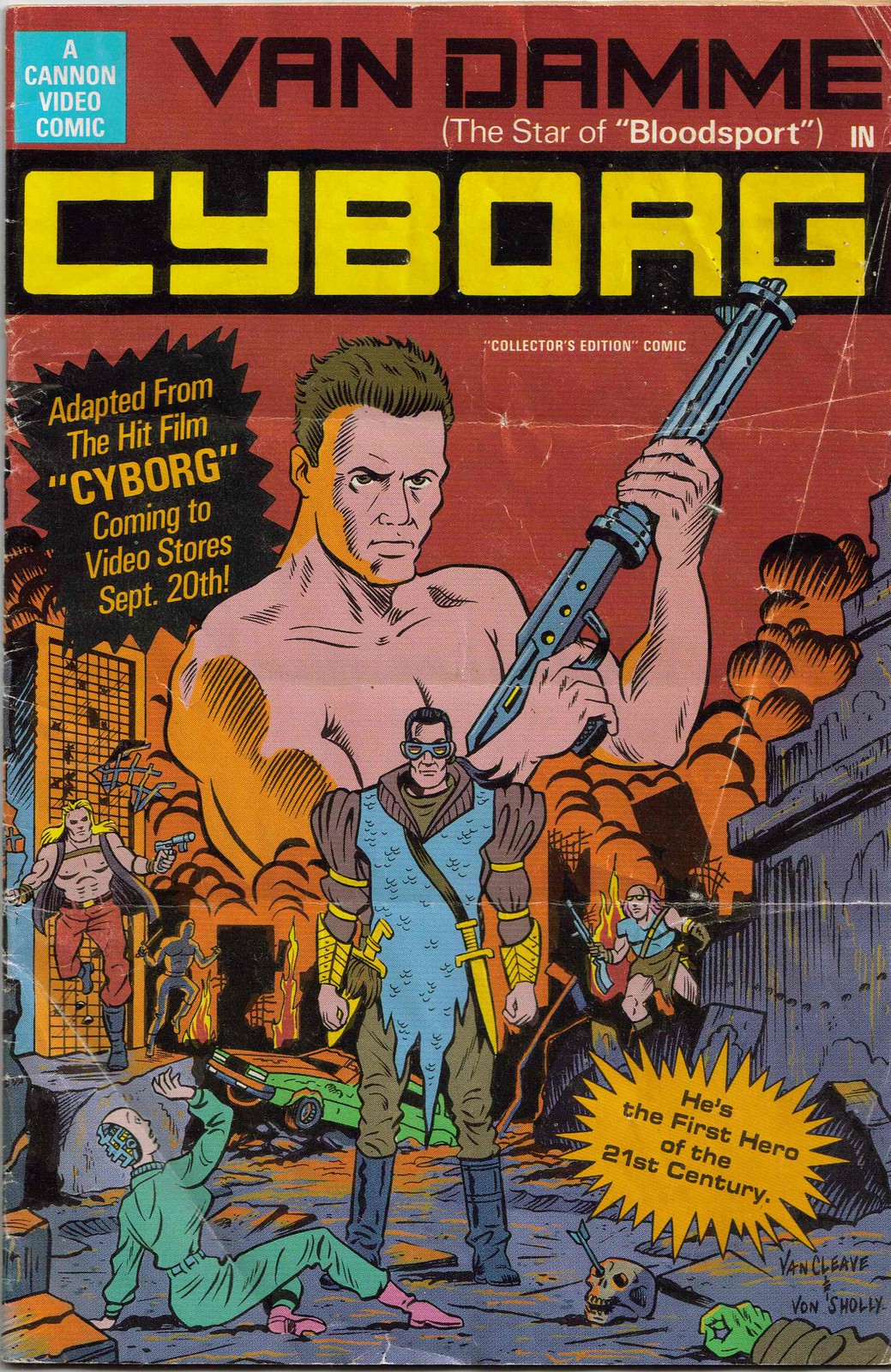The image depicts a highly detailed, vintage comic book cover titled "Van Damme Cyborg." Dominated by a red background, the scene captures an action-packed, apocalyptic cityscape with destroyed buildings, fire, and chaos. Front and center is a shirtless Jean-Claude Van Damme, armed with a massive futuristic gun. He dons ragged chainmail, gold gauntlets, dark green pants, and black boots. To his side are two small dagger swords holstered at his belt. In the background stands a war-torn green car and a bald figure in a green jumpsuit with pink boots, revealing robotic insides from a damaged head, appearing fearful of Van Damme. Additional characters are visible, such as a man in a yellow and blue face mask and another with red pants, contributing to the chaotic ambiance. Text on the cover reads "Van Damme, the star of Bloodsport - Cyborg," promoting its adaptation from the hit film "Cyborg," with a release date of September 20th for video stores. Labeled as a Canon Video Comic, this collector's edition is hyped as featuring the first hero of the 21st century. The creators, Van Cleave and Von Sholly, are noted at the bottom.